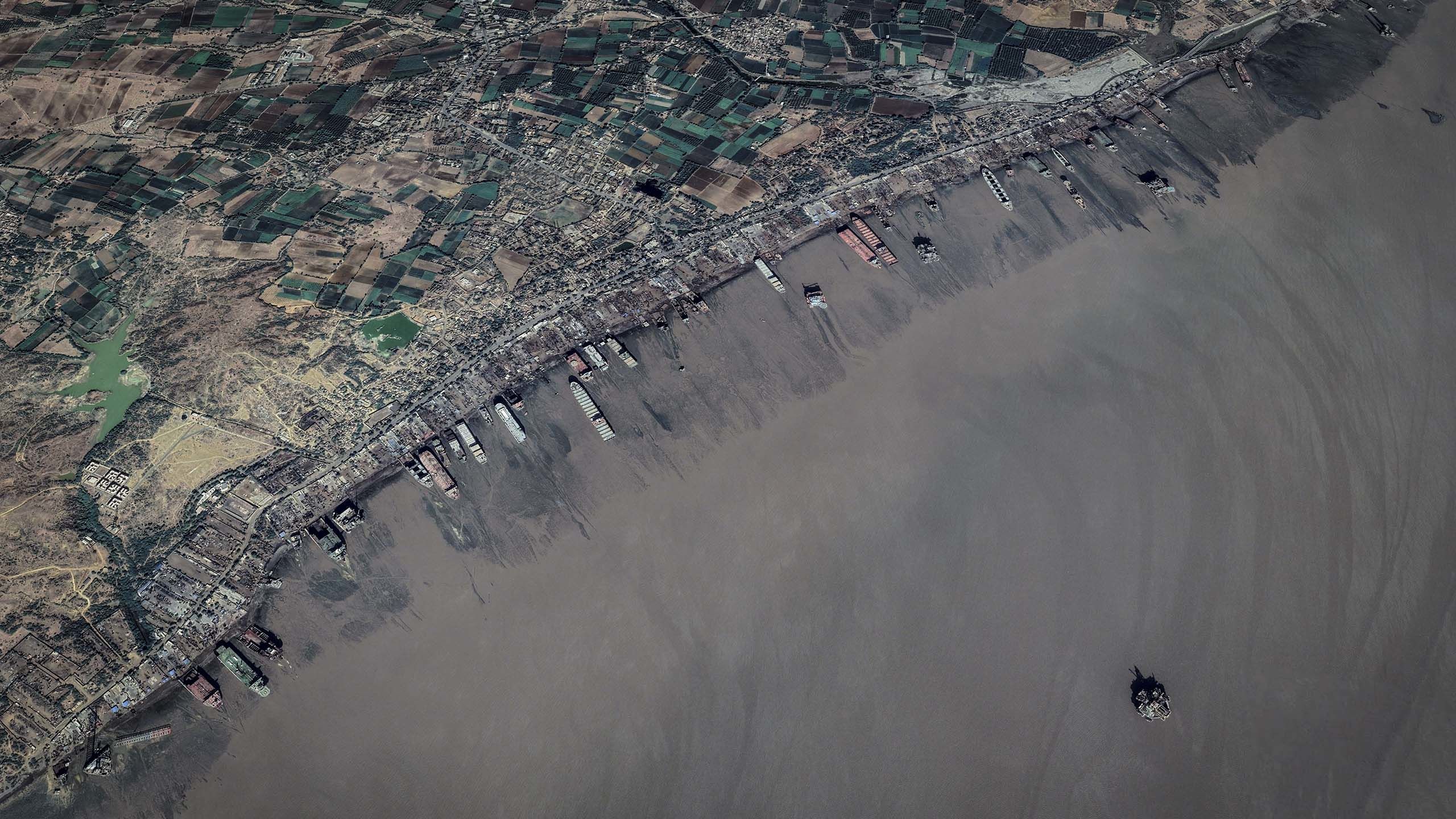The image presents a rectangular aerial view of a coastal and tidal area, characterized by a drab and murky landscape. On the left-hand side of the picture, there is land with scattered patches of green and brown, interspersed with numerous small buildings, giving the impression of dots from the sky. A road is visible cutting through this landscape. Progressing from the bottom left to the upper right, the image reveals a shoreline where a series of boats are parked, which may appear to be docked along the shore or perhaps stranded in a tidal area during low tide, exposing a vast mudflat. The water is notably gray and swirling, indicating a very dark, muddy, and murky appearance. The marina area shows a concentration of boats, and the water color ranges from grayer near the shore to varying shades of gray with darker swirls further out. There is a black, round object - possibly a buoy - floating in the water, with a hint of grayish tan underneath it. The overall scene is quite muted and lacks vibrant colors, contributing to its dull and lifeless aesthetic.